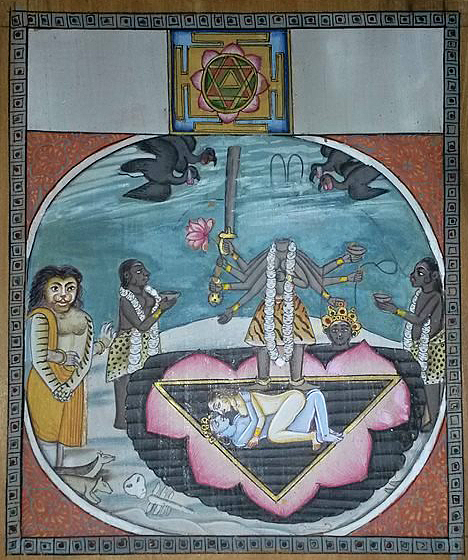The image portrays a richly detailed painting or illustration of Hindu gods and goddesses. Dominating the center is a decapitated deity figure, drawn in grey, with multiple arms. This figure is holding their own severed head in one hand and various weapons, including a sword, in the others. The deity is adorned with a brown leopard print skirt and a necklace of skulls, famously depicting aspects of divinity and mortality. Additionally, the deity holds a pink lotus flower, symbolizing purity and spiritual awakening.

Flanked on either side of the central figure are two disciples, depicted in similar attire, offering prayers. To the left stands a priest-like figure dressed in an orange outfit, adding to the religious ambiance. Above, at the top of the illustration, grey vultures drink from a blue cloud, an unusual yet symbolic element enhancing the mystic atmosphere.

Below, a triangular inset showcases an intimate scene reminiscent of Kama Sutra art, featuring a blue-skinned deity and a fair-skinned woman entwined in an embrace against a pink background. This triangular section adds layers of complexity and depth to the artwork.

At the top center of the image is a Yantra design enclosed in a golden square, marked by a circular pattern with a star and pink flower petals, symbolizing spiritual geometry. The entire painting is framed by a detailed border of grey and black squares with central dots, enclosed further by an orange outer border, encapsulating the intricate Hindu stylistic elements.